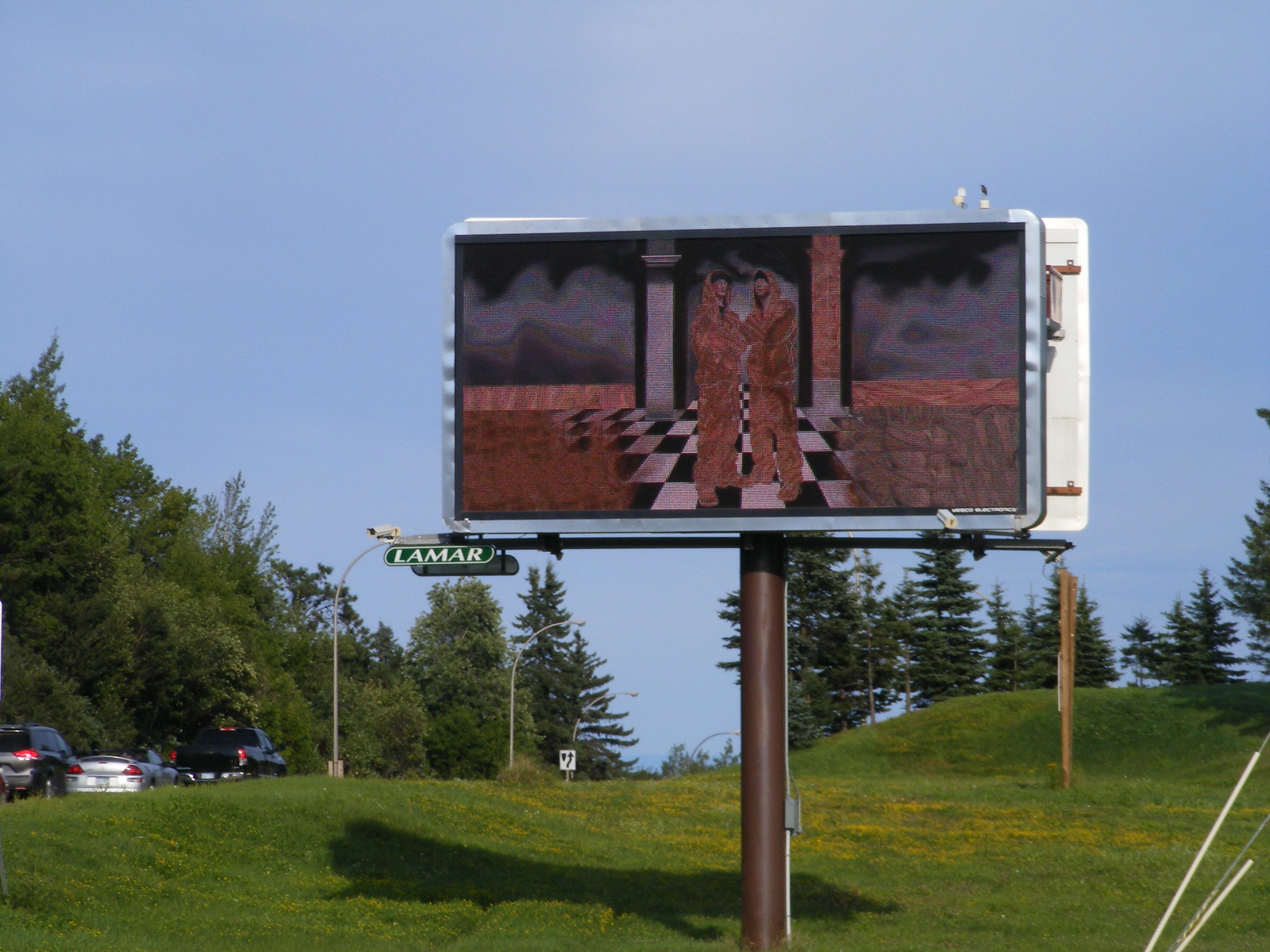In this picturesque scene, a prominent billboard immediately catches the eye. The billboard, set amidst a lush, green grassy expanse, depicts two hand-drawn male figures in matching brown sweatsuits, standing on a black and white checkered tile floor with their arms crossed. Their faceless outlines give them an enigmatic air. Surrounding this central image, large trees line the roadside, adding to the natural beauty of the area. On the left side of the image, a road curves northward, with three cars visible, traveling along this route. Adding a layer of intrigue, a street sign marked "Lamar" stands adjacent to the billboard, equipped with a camera, suggesting a monitored or well-traveled area. The juxtaposition of natural elements with urban signage creates a captivating and serene setting.